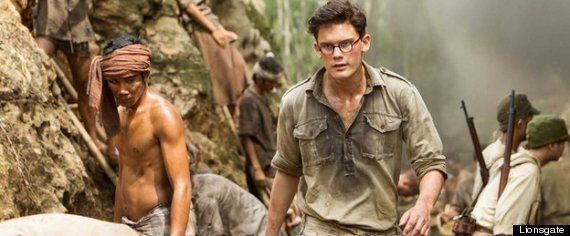This image appears to be a movie still, indicated by the "Lionsgate" logo on the bottom right. Central to the scene is a young man in his 20s, with brown hair and glasses, wearing a light green short-sleeved button-down shirt that is soaked in sweat. He looks highly focused and possibly distressed, suggesting he's navigating a tense or dangerous situation. To his right, there's a bare-chested, tan-skinned, Asian man with a peach-colored scarf tied around his head, standing near a large tree trunk. In the far right background, two individuals dressed in white shirts and khaki army caps are visible, carrying rifles on their backs. The backdrop includes smoke and some trees, adding to the war-torn atmosphere of the scene. The bottom left of the image also features a small "Mangia" insignia, possibly denoting another production detail.